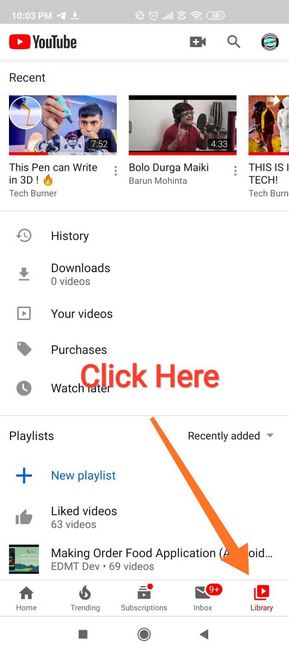The image depicts a vertical rectangular page from a YouTube mobile interface. At the top of the page is a gray header bar displaying the time "10:03 p.m." in white text. Directly below this, the YouTube logo and the word "YouTube" are prominently displayed. Below the logo, the word "Recent" indicates the section for recently watched or suggested videos.

The first video thumbnail features a man holding a pen, and the title below the thumbnail reads "This Pen Can Write in 3D - Tech Burner". Adjacent to this thumbnail, the second video features a person dressed in red, with the title "Bolo Derga Mekai - Baron Mohinta" below it. On the far right, another partially cut-off thumbnail shows some standing people, with the title "This is Tech - Tech Burn" below it.

Beneath the thumbnails, a row of navigation icons is displayed, starting with a circle containing a clock icon labeled "History". Next is an arrow pointing downward over a horizontal line, labeled "Downloads - 0 videos". Following this, an icon of a square with an arrow pointing to the right is labeled "Your Videos". Below this is an icon of a price tag, with the text "Purchases", and next to it, a clock icon with the text "Watch Later".

Lower down, the text "Playlist" is followed by "Recently Added" and "New Playlist", along with "Liked Videos, Making Order Food Application".

At the bottom of the page, a row of icons provides quick access to various sections of the YouTube app: 'Home', 'Trending', 'Subscriptions', 'Inbox', and 'Library'.